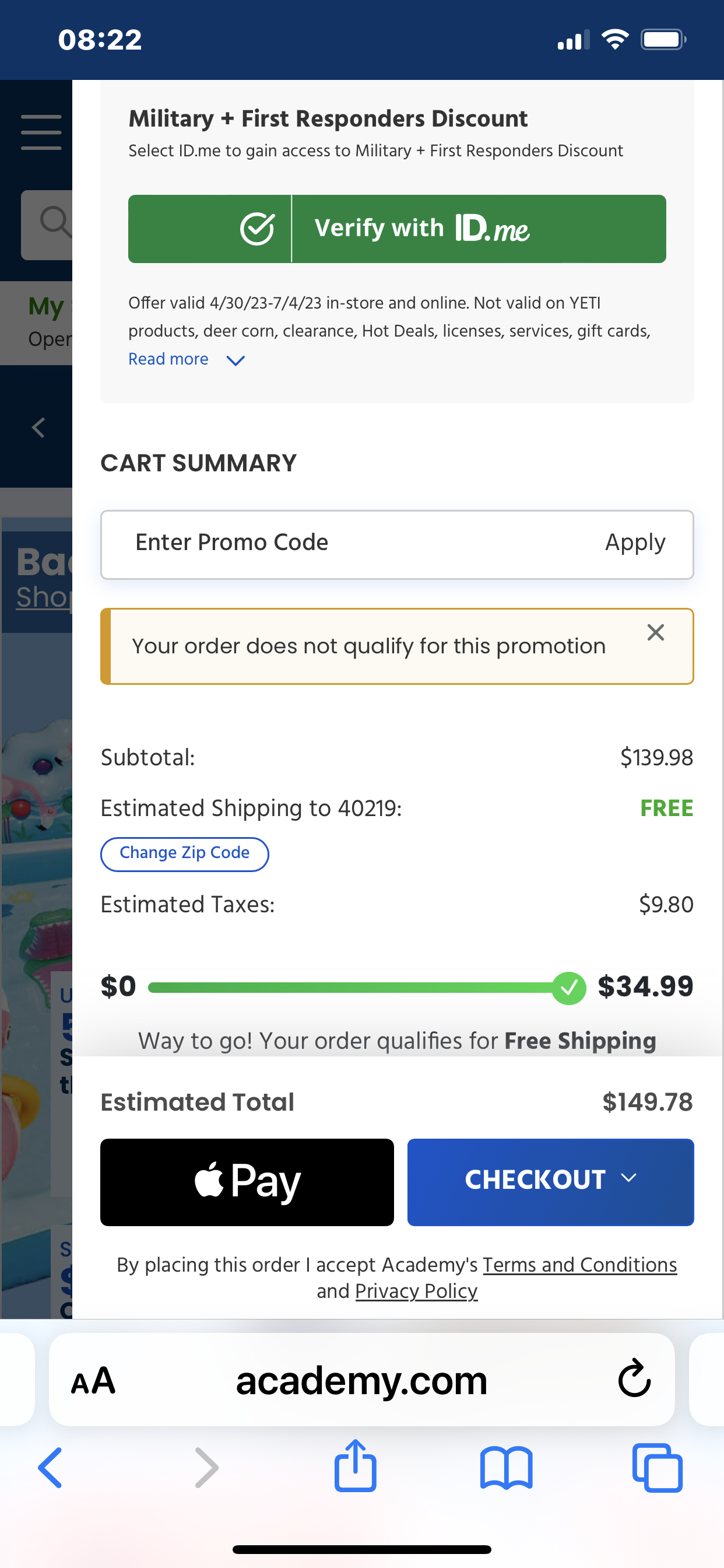The image is a vertically elongated screenshot, approximately three times as high as it is wide, taken from a cell phone. At the very top, occupying the top 5% of the image, there is a dark blue background featuring white text on the left displaying the time as "08:22". On the right side, icons show three out of four bars for Wi-Fi signal, full cellular signal strength, and a mostly full battery indicator.

The main focus of the image is a window on the right, taking up roughly 85% of the width. This window has a white background. To the left, a dimmed background occupies the remaining 15%, suggesting a layered interface.

At the top of the white window, the text "Military + First Responders Discount" is prominently displayed in black. Below this text, there is a smaller line of details. A dark green button follows, filled with a white check mark on the left and the text "Verify with ID.me" extending to the right. Beneath this green button, a three-line disclaimer is presented in a very small font.

About one-third of the way down the image is a section labeled "Cart Summary". This section includes a box for entering a promo code. Just below this, there is a mustard yellow-bordered box with black text inside, stating "Your order does not qualify for this promotion."

Towards the bottom of the white window, the subtotal is listed as "$139.98", and the estimated shipping cost is highlighted in green text as "Free".